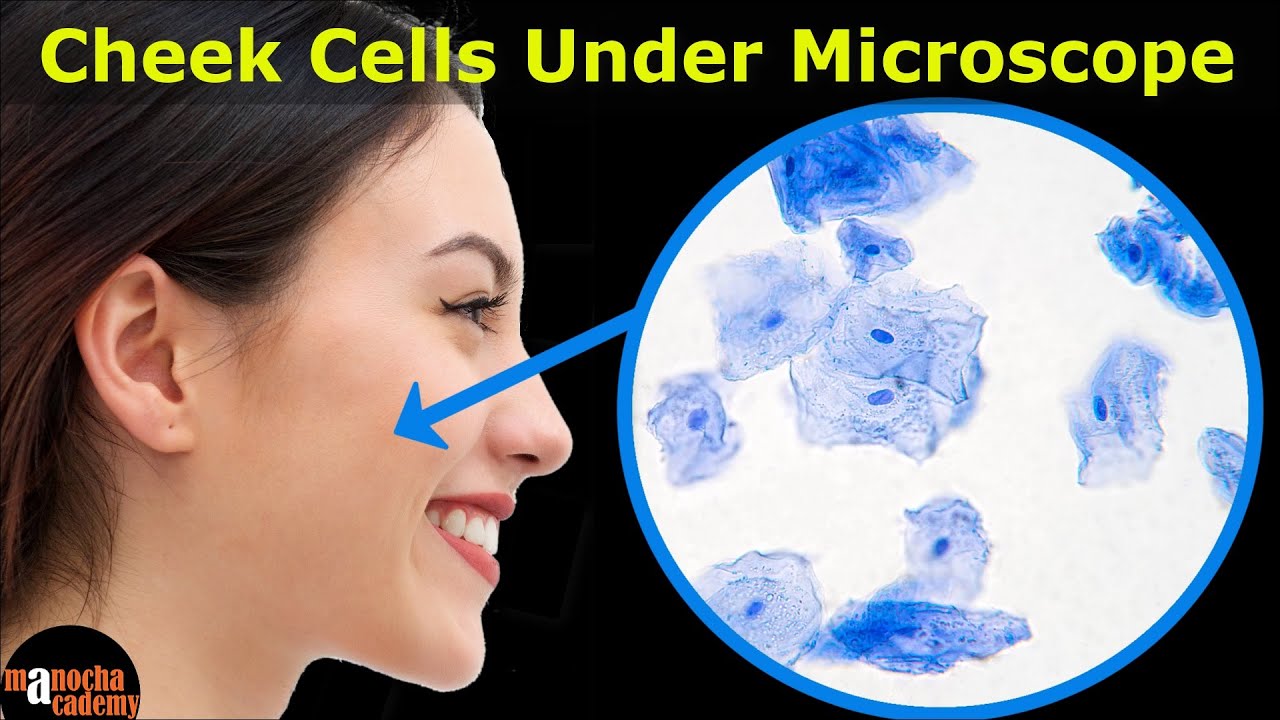This YouTube thumbnail features an image of Congresswoman Alexandria Ocasio-Cortez, who is of light complexion with brown hair, smiling and looking toward the right. The background is black. At the top, the title "Cheek Cells Under Microscope" is written in yellow letters. An arrow points from her cheek to a zoomed-in view of her cheek cells, depicted within a blue circle. The cells are irregularly shaped, resembling crumpled rectangles or paper bags; they are mostly light blue with dark blue ovals in the center. In the bottom left corner, the text "Minoka Academy" is displayed inside a black circle, with the letters mostly in orange except for the 'A,' which is white.